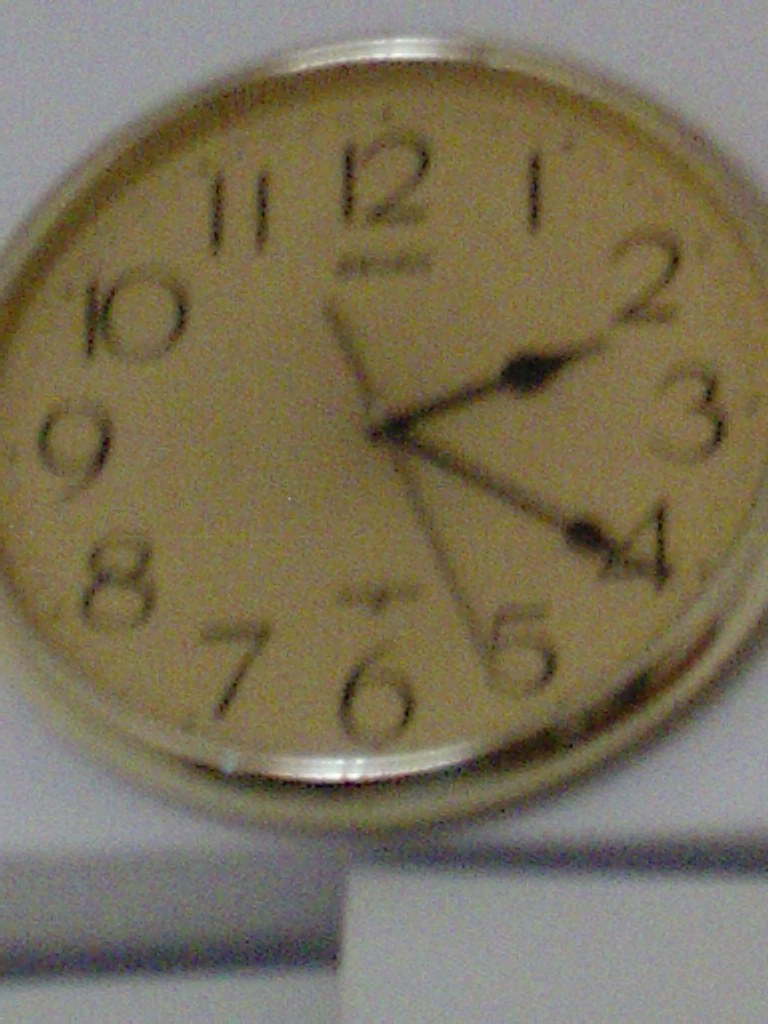This is a blurry digital photograph of a circular wall clock mounted on a white wall. The clock has a silver metal trim and an off-white face that appears yellowish in the image, likely due to distortion. All the numbers from 1 to 12 are clearly visible around the clock's face. The hour and minute hands are thin and black with bulbous tips, and there is a black second hand, currently pointing at around 21 seconds past the minute. The time on the clock reads approximately 2:21. Some text is present underneath the 12, but it is too blurred to read. The background is uniformly white, with a possible doorway located in the bottom quarter of the image, identifiable by a black slit above what seems to be two white panels. The scene suggests a simple, modern setting, possibly an office or a school, with no additional text or people visible.